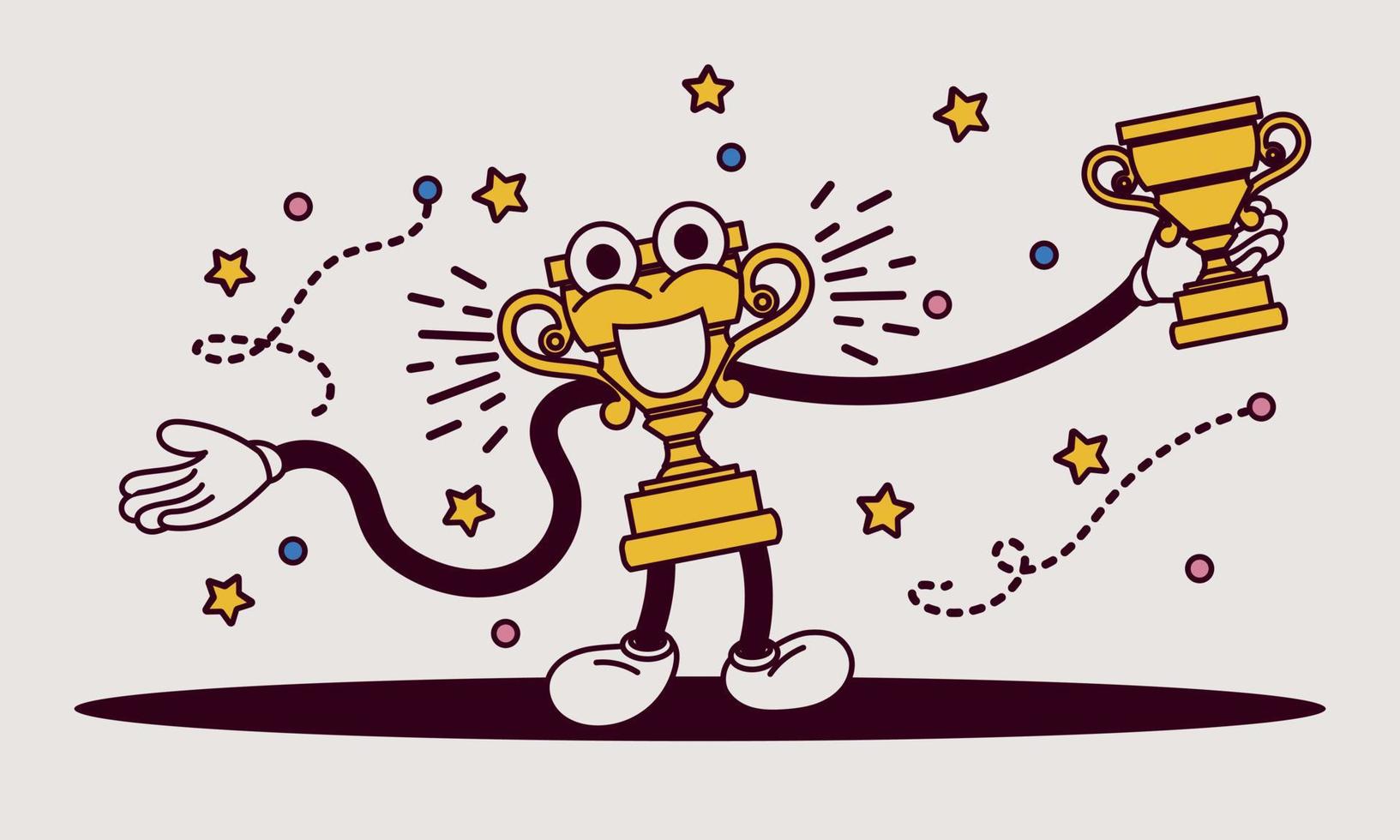This detailed, descriptive caption combines elements from all three source captions:

A graphic illustration depicts a whimsical cartoon character with a body shaped like a trophy. The character has two handles on its sides serving as ears, along with large eyes on top and a smiling mouth in the middle. The base of the trophy mimics hips, transitioning upward into a neck and arms. Its arms have hands donned in white gloves, while its legs and feet resemble Mickey Mouse's iconic shoes. A circle, presumably its shadow, lies beneath the character on a plain gray background. Adding to its playful design, the character holds a miniature trophy in its left hand that mirrors its own trophy-like form. Surrounding the character are vibrant yellow stars, red and blue circles, with dotted lines connecting them, creating a dynamic trail effect that gives the appearance of movement in the abstract backdrop.